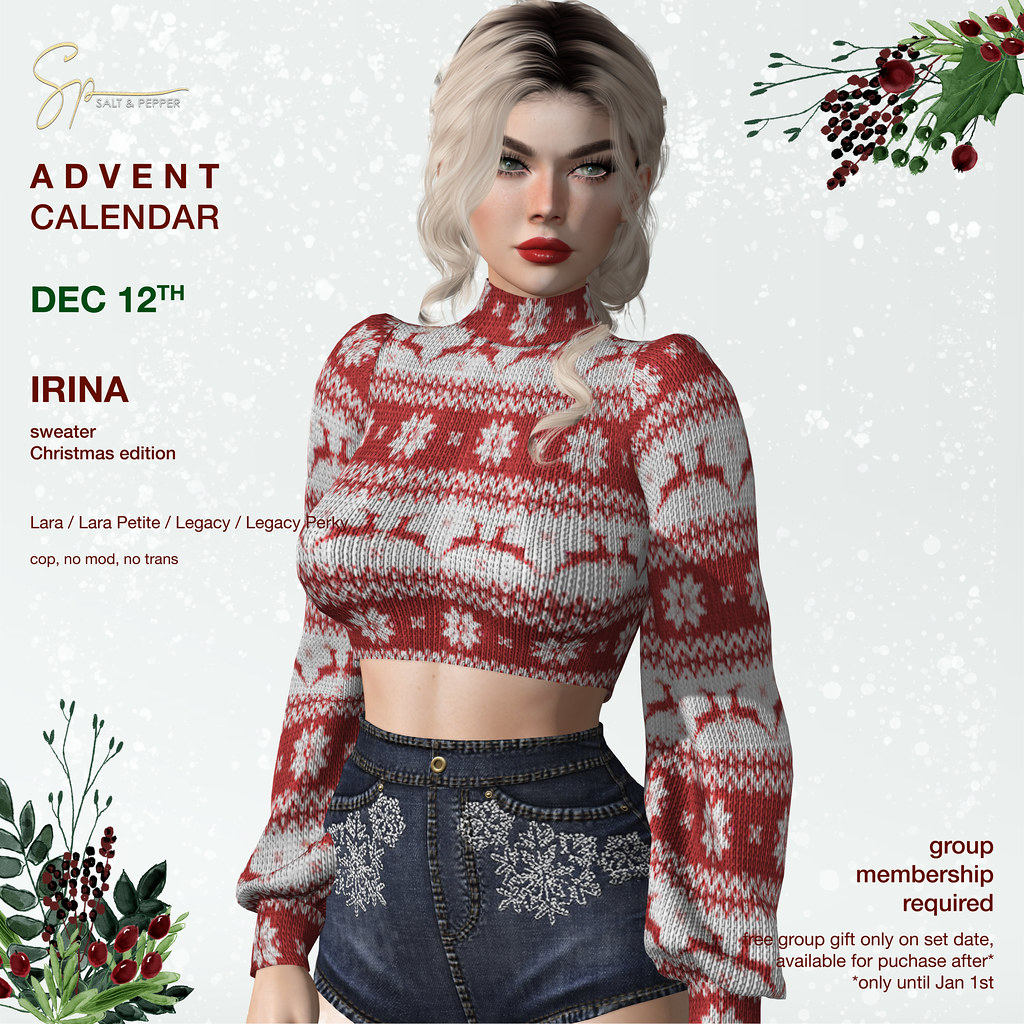This image is a detailed square-shaped, digitally illustrated advertisement with a Christmas theme. It features a wintery, light-blue background adorned with small white dots resembling snowflakes, complemented by festive holly sprigs in the upper right and lower left corners. The central figure is a heavily made-up young woman with strikingly whitish-blonde hair styled in ringlets. She exudes a doll-like appearance and wears a high-neck, red-and-white cropped sweater with long sleeves that showcase Christmas motifs, including snowflakes and reindeers. Her midriff is exposed, and she pairs the sweater with short, dark denim shorts embroidered with snowflake patterns on the pockets. The overall composition lends a sense of festive charm through its combination of illustration and graphic design elements.

Text on the advertisement includes: "Salt and Pepper Advent Calendar December 12th Irina Sweater Christmas Edition Lara Lara Petit Legacy Legacy. Group membership required. See group gift only on set date available for purchase after only until January 1st." Additional details state "Perky, Cop, No Mod, No Trans," indicating the exclusivity and special conditions associated with the featured items.